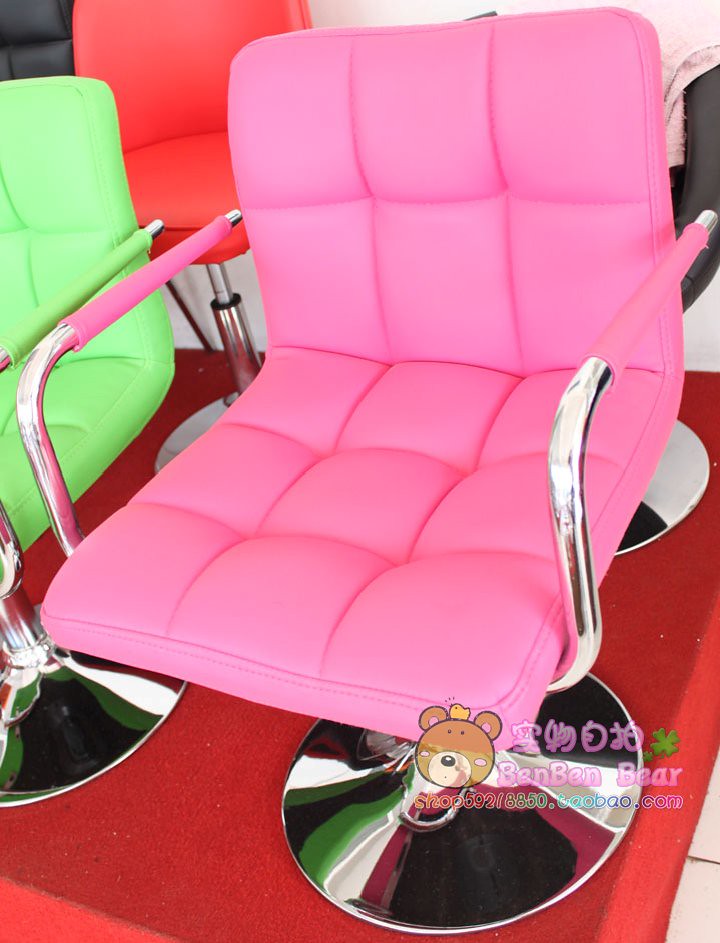This close-up photo, likely an advertisement, features an array of colorful chairs displayed in a shop or marketplace setting. The main focus is a plush, bright carnation pink chair with a button-patterned leather upholstery. The chair is designed to appear very comfortable, possibly functioning as a barber chair, with a silver, swiveling base. It has curved silver arms covered with matching pink leather pads. Positioned on a red podium, the chair is flanked by a neon lime green chair and a bright coral chair in the background. Additionally, the image includes the logo "Ben Ben Bear" in the lower right-hand corner, along with a small bear icon and a partially visible website URL. This logo suggests it might be the brand or owner of the image. The overall composition is slightly imperfect with some cropping issues, but it highlights the vibrant seating options and the shop's playful aesthetic.